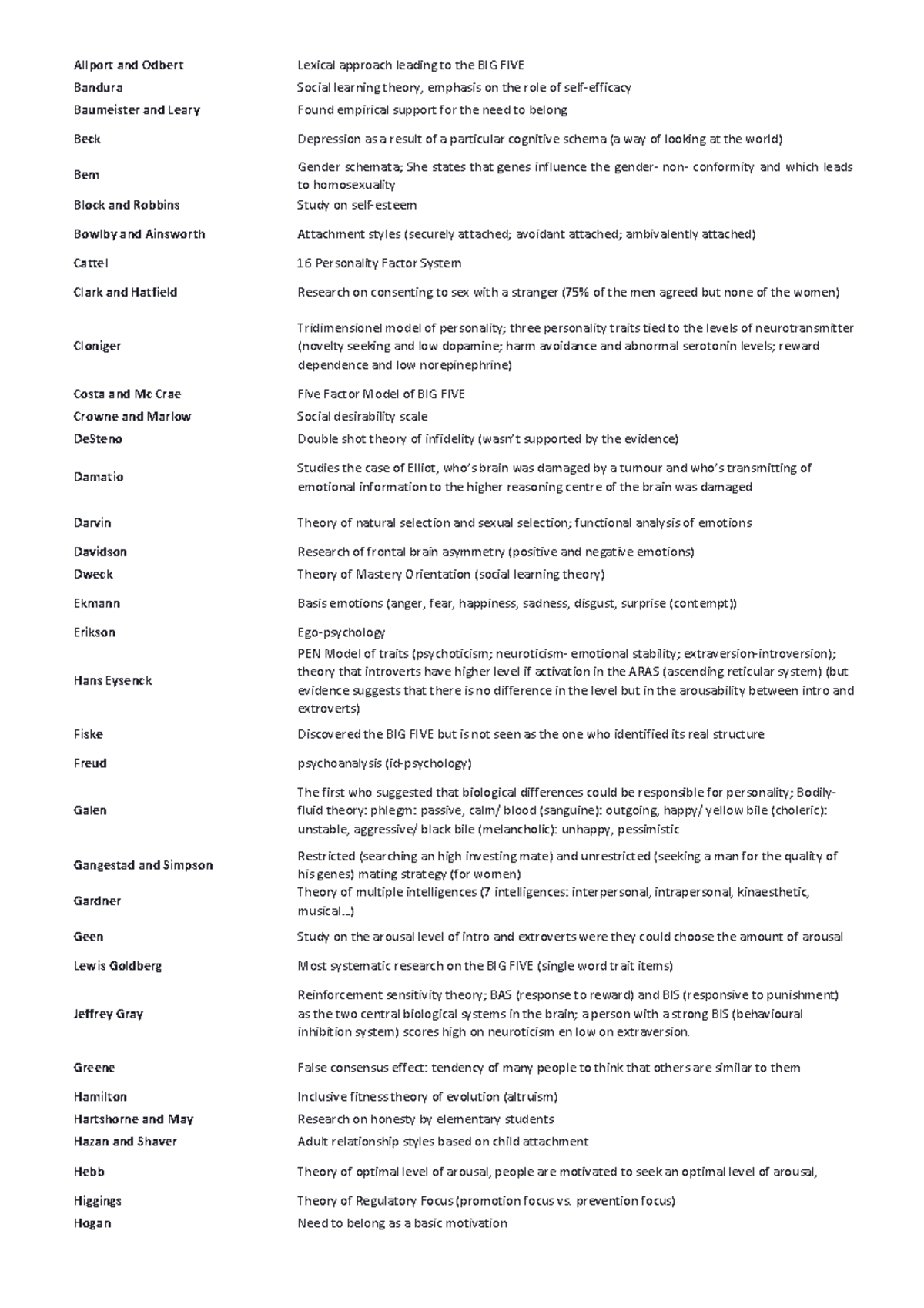The image appears to be a screenshot of a text-based document, displaying a collection of psychological theories and key concepts. On the left side of the image, there are names of various psychologists and theorists, while on the right side, brief descriptions of their theories or findings are provided. The first entry mentions Allport and Odbert, followed by a description of the lexical approach leading to the Big Five personality traits. It then highlights Bandura's social learning theory, which emphasizes the role of self-efficacy. Another entry attributes Baumeister and Leary with empirical support for the need to belong. Beck is noted for linking depression to certain cognitive schemas or ways of viewing the world. Ekman's basic emotions—anger, fear, happiness, sadness, disgust, and surprise—are mentioned, along with the addition of contempt. Erickson is associated with ego psychology, and Freud with psychoanalysis. The final entry discusses Hogan's assertion that the need to belong is a fundamental motivation.